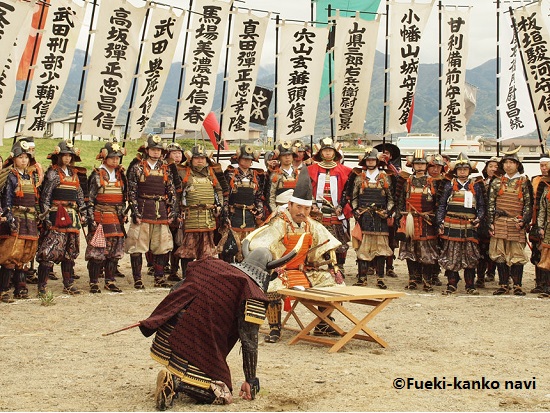This photograph, potentially taken in Asia, captures a scene reminiscent of a historical or ceremonial re-enactment involving individuals dressed in traditional samurai armor. They are situated outdoors on a light tan dirt ground. The central focus is a man in elaborate attire, wearing an orange and gold samurai outfit with a black hat, seated at a small light-colored wooden table. Kneeling before him is another individual clad in a burgundy cloth draped over his shoulders and a striking black helmet adorned with large, horn-like protrusions. Surrounding them are approximately 20 other participants dressed in samurai armor, all featuring different helmets with various gold insignias. The background is adorned with numerous tall white flags displaying Japanese writing, adding to the ceremonial ambiance. The scene, which bears a copyright notice from 'FUEKI-KAN-KO-NAVI' in the bottom right corner, suggests a meticulously staged event, possibly for a film or traditional reenactment.